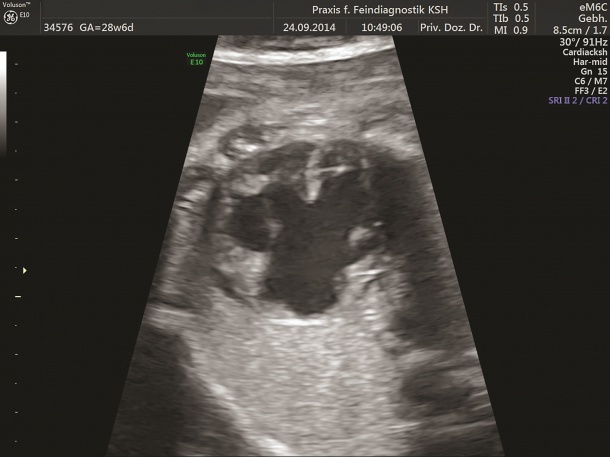This image is a grayscale sonogram, marked with text in what appears to be German. It says "Praxis F. Fine Diagnostic KSH," suggesting a specialized diagnostic practice. The sonogram measures some parameters, notably "8.5 cm / 1.7" and angles such as "30 degrees". The text "Cardia CKSH" appears, hinting that it might be a cardiac ultrasound. 
The image itself is predominantly black with varying shades of gray. It's ambiguous and unclear, as it doesn't distinctly show a human form typical of prenatal ultrasounds, but rather a central blackish-grayish blob flanked by two lights in a triangular, spotlight-like shape. The top section of the image has a gray bar displaying several measurements and acronyms, presumably medical metrics, while additional details are in the top right corner. These details include technical terms and numbers, such as "HR-MID, GN15, C6-M7, FF3-E2." The entire image seems diagnostic in nature, primarily focused on displaying internal measurements rather than a clear anatomical figure.